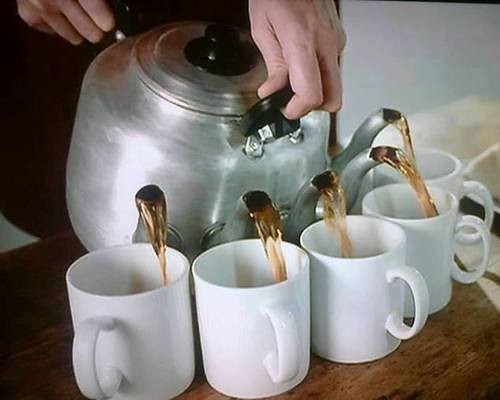The photograph captures a unique and intriguing scene of a stainless steel or aluminum teapot with five spouts, simultaneously pouring a light brown liquid, possibly coffee or tea, into five white porcelain mugs. The teapot is shiny, reflecting light, and features two black plastic handles—one in the front and one at the back, along with a black knob on its metal lid. The person pouring, whose hands are visible, is dressed in a dark apron with white pants, and slightly leans forward while holding the pot. The five mugs are meticulously arranged in a half-moon or arc shape on a brown wooden surface that shows a distinct wood grain. The handles of the mugs are pointing outward. In the background, there are hints of a white tablecloth or napkins, and a light-colored floor, which adds to the cozy indoor setting of this intriguing image.